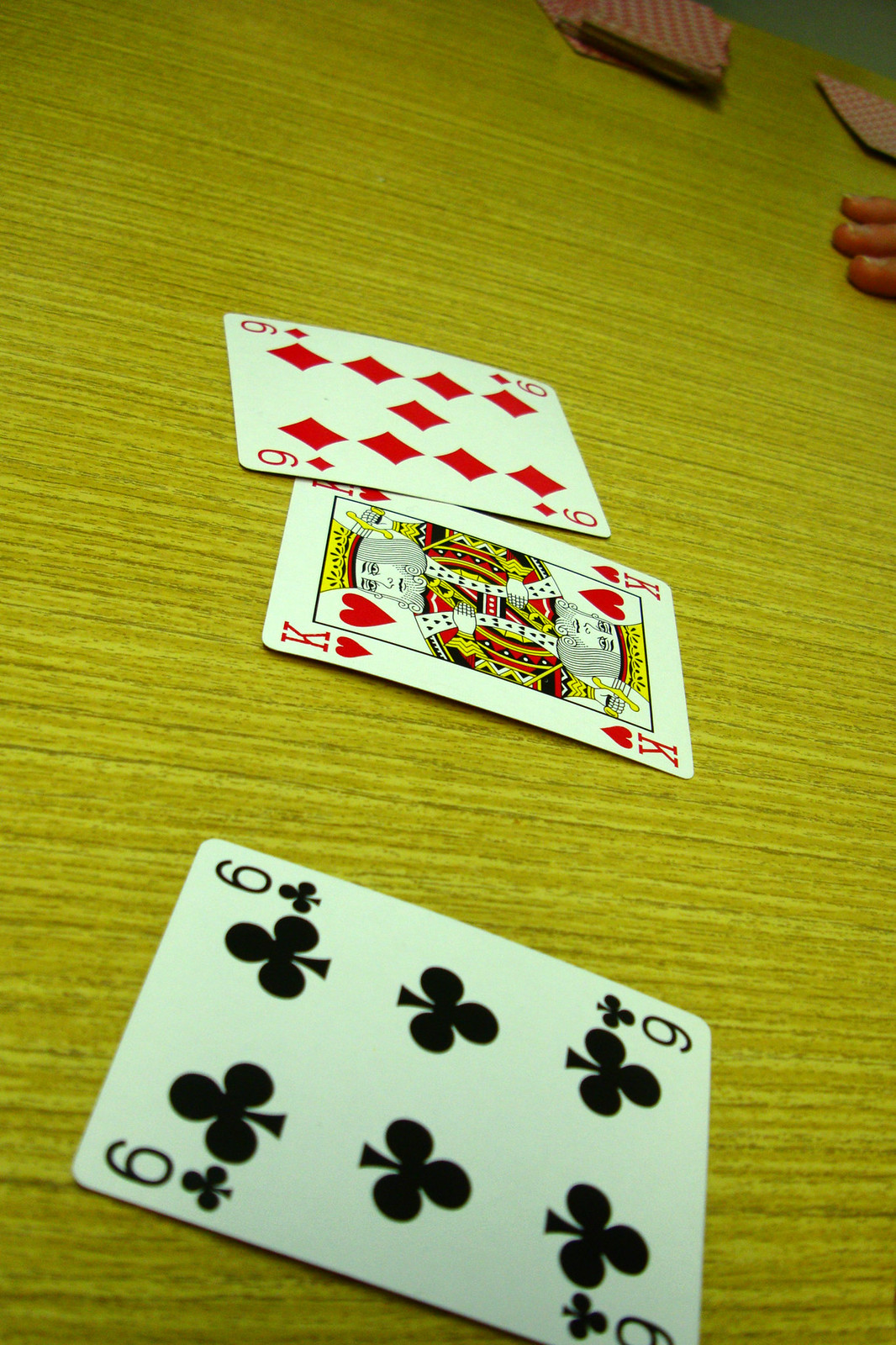In the photograph, a close-up view of playing cards is displayed on a finely grained, slanted wooden table. The six of clubs, prominently featured in the foreground, captures immediate attention with its bold black symbols. Positioned centrally is the king of hearts, its vivid red color standing out distinctly. Furthest back, the nine of diamonds adds another splash of red to the composition. To the right edge of the image, partial fingers and fingernails of a person are visible, delicately touching the cards. In the background, a neat stack of additional cards can be seen, hinting at an ongoing game or arrangement. The rich texture of the wooden surface beneath the cards enhances the overall visual appeal of the scene.